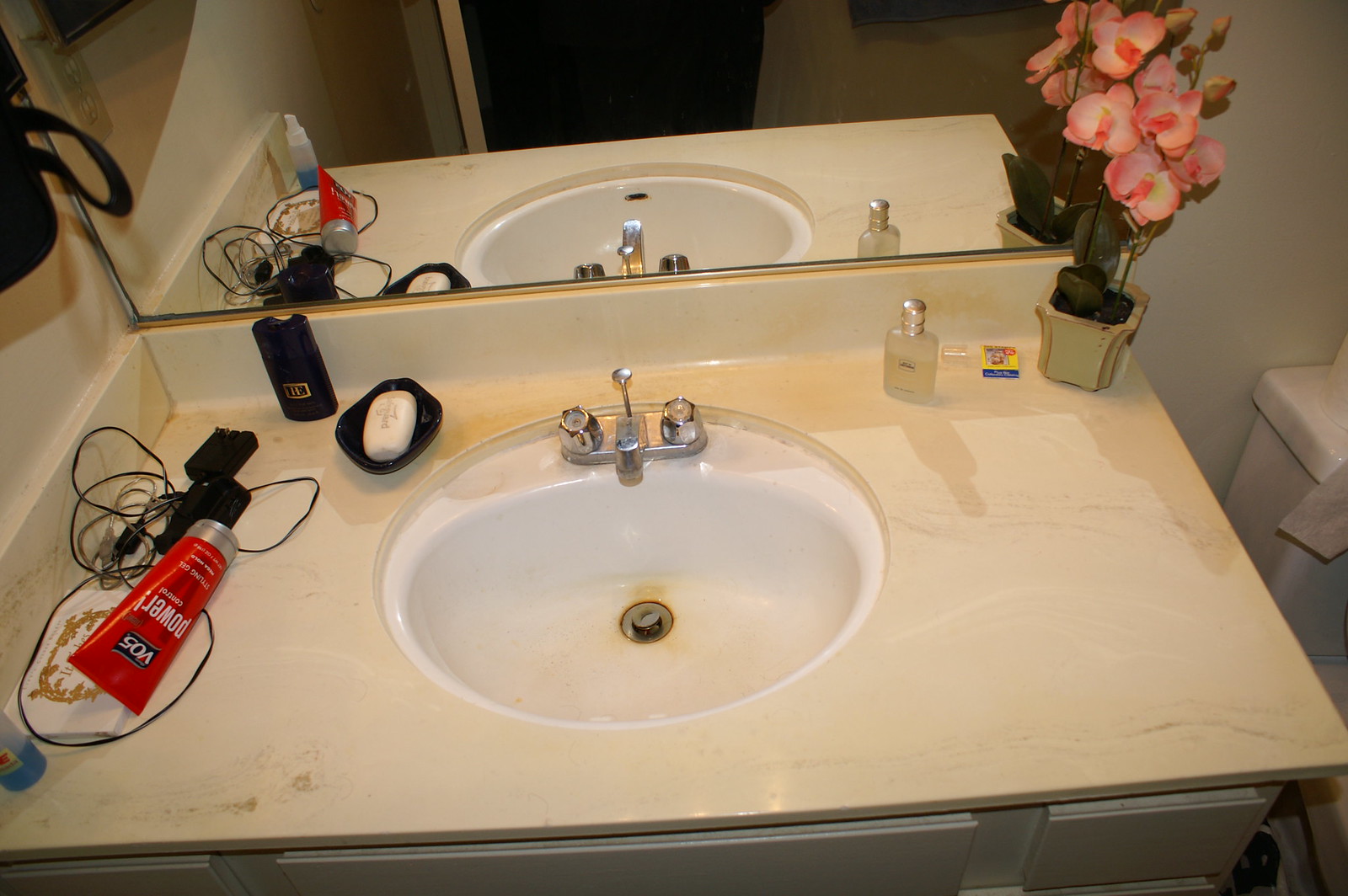This photograph depicts a pristine white countertop with a central white sink, which shows slight rusting around the drain. The sink is flanked by a silver faucet and matching silver handles. Below the countertop, white drawers complement the clean aesthetic. The backdrop of the image is a stark white wall, enhancing the overall sense of cleanliness.

On the countertop, a clear jar holding vibrant pink flowers brings a splash of color. Nearby, a black soap dish houses a white bar of soap, and next to this, there is an unidentified brown object. Adding to the array of items, a red tube labeled "VO5" stands out, and an electrical appliance with a visible cord adds a touch of modern utility. Above the counter hangs a mirror, perfectly reflecting the sink and countertop setup.

To the right edge of the picture, the top of a white toilet is partially visible, further indicating that this is a bright, utilitarian bathroom space.